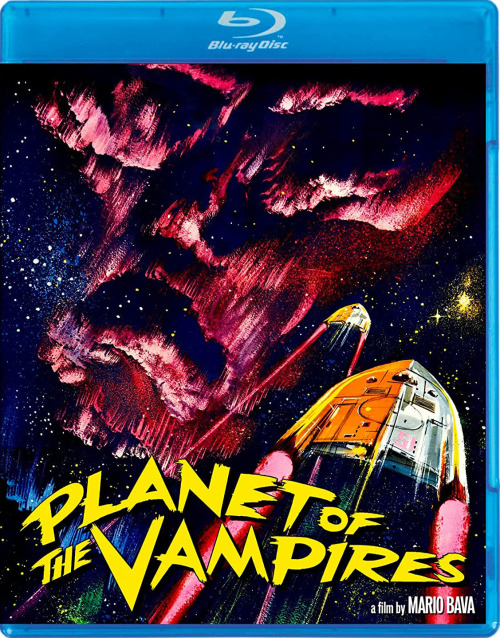This is the cover of a Blu-ray disc for the movie "Planet of the Vampires," directed by Mario Bava. The background is dark, featuring a cosmic scene with various stars in yellow and white. Dominating the cover is a large, red, skull-like face embedded within the stars, giving an eerie and dramatic effect. In the lower right corner, there is a rocket ship blasting off into space, accompanied by a smaller spaceship. The scene also includes aurora-like red and pink clouds, enhancing the celestial ambiance. The title "Planet of the Vampires" is prominently displayed in a futuristic, yellow font, and the Blu-ray logo is positioned at the very top of the image.